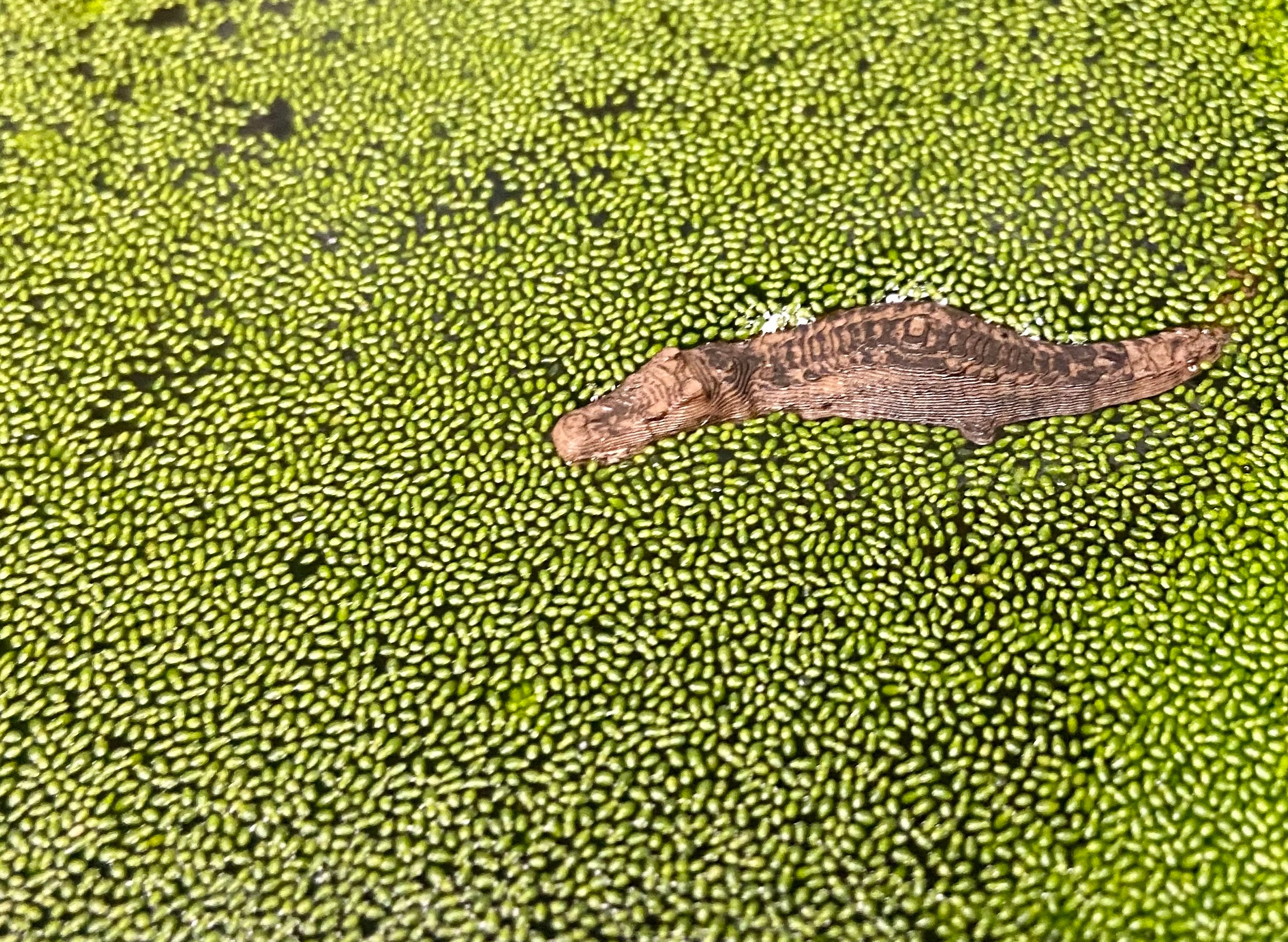This outdoor photograph captures a textured and intriguing scene of a brown alligator or crocodile amidst a pond covered with dense green vegetation. The water itself is barely visible, obscured almost entirely by what appears to be a layer of round green pellets or large green peas, giving the pond a visually striking, ball-pit-like appearance. The sparse gaps in the green covering reveal small patches of gray water underneath. The alligator, with its light to dark brown coloration and distinctive markings along its back, glides through the water, with parts of its tail submerged and its legs mostly hidden. The creature's face is tan around the mouth, and its snout has a blunt, less pointed shape. The overall image is devoid of text or human presence, highlighting the natural, almost surreal environment.